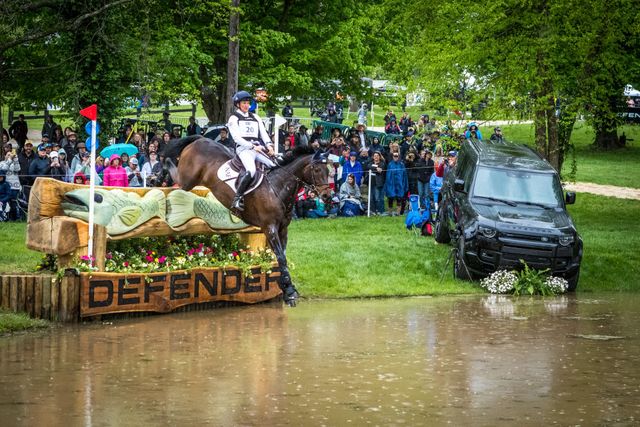The photograph captures a dynamic outdoor scene during the day, featuring a horizontally oriented landscape. In the foreground, a broad expanse of shallow, brownish water—possibly a pond—occupies the bottom quarter of the image. Towards the center-left, a notable wooden structure bearing a sign with the word "Defender" stands prominently. This structure is adorned with carved fish and surrounded by flowers. A woman, attired in a full jockey outfit with a helmet and a numbered chest plate, is astride a dark brown horse with a black mane; they appear to be in mid-jump over the Defender sign, leaping towards the water.

To the right of this action, almost at the water's edge, a jeep-type vehicle is precariously positioned, as if on the verge of driving into the pond. The scene's background features lush grass and a dense line of green trees, behind which stands a sizable, tightly-packed crowd of approximately 50 to 100 onlookers. Some crowd members are equipped with rain gear and umbrellas, suggesting an impending or ongoing drizzle. This lively scene, with its blend of spectators, natural elements, and the intense moment of the horse and rider's leap, creates a vivid depiction of an equestrian event.